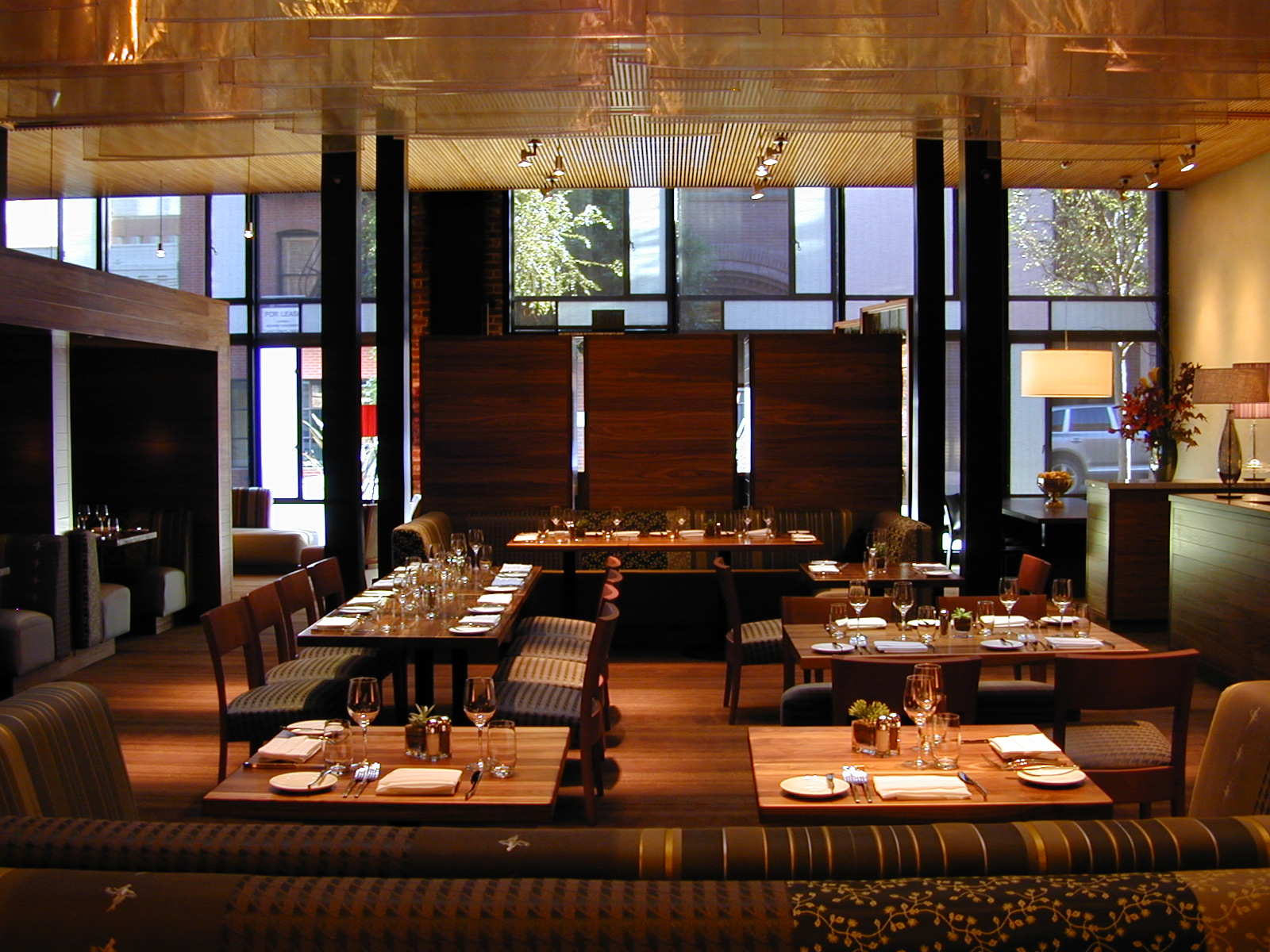This color photograph captures the warm, inviting interior of an empty fine dining restaurant. In the foreground, there are two small, square wooden tables, each set for two people with white plates, clear wine glasses, forks, napkins, and small plants. These tables are accompanied by wooden benches. Further into the room, additional longer wooden tables are visible. The table to the left is arranged vertically and set for eight people, while the one to the right is set horizontally for four people. Both tables feature similar settings with plates, wine glasses, and plants. Another table can be seen along the back wall, though its exact capacity is unclear. The chairs around these tables have wooden backs and cushions with white and gray stripes. On the far left, a series of cozy booths offer alternative seating options. To the far right is a desk area, likely serving as the register for paying. Large windows in the background allow a glimpse of parked cars, a street, and the green foliage of trees outside, imparting a serene atmosphere enhanced by the light blue tint of some windows and the warm-toned indoor lighting. Three large wooden panels near the back wall appear to serve as a room divider.